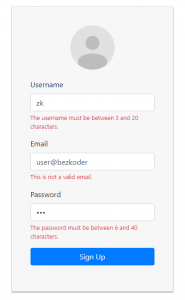This is a detailed screenshot of a sign-in page predominantly shaded in gray. At the top center of the page, there is a circular icon featuring a grayed-out silhouette placeholder for a profile picture or avatar. Below this, there is a text field labeled "Username" with the entry "ZK" already filled in. A red error message underneath the username input reads, "The username must be between 3 and 20 characters."

Further down, there is another labeled text field for "Email" where the currently entered address is "user@B-E-Z-K-O-D-E-R." A red warning message below indicates, "This is not a valid email."

The third text field on the page is labeled "Password," with three characters entered. Below this field, another red error message states, "The password must be between 6 and 40 characters."

At the very bottom of the page, there is a prominent blue rectangular button with the text "Sign Up" in white font.